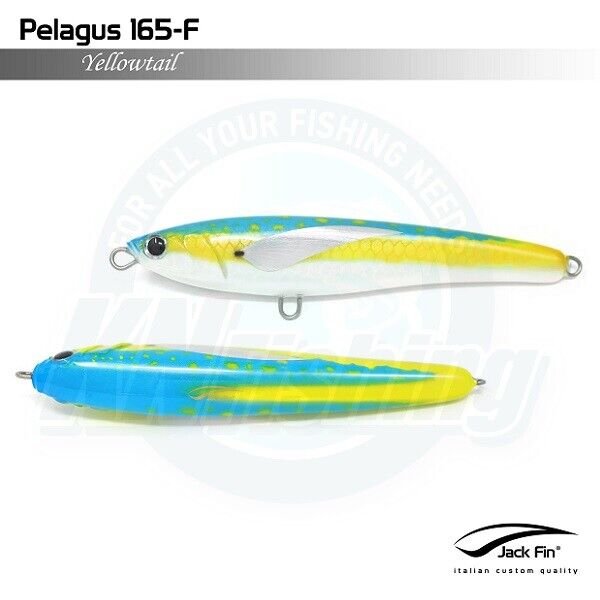The image is an advertisement for a fishing lure, displayed within a light blue rectangular frame that is shorter on the left and right sides than it is on the top and bottom. At the upper left corner, the text "Pelagos 165-F" is written in a dark gray, slightly squished font. Beneath this is a horizontal banner that fades from black on the left to almost white on the right, containing the italicized, capitalized text "Yellowtail" in smaller, white typewriter font.

Centered in the middle of the image, superimposed over a faded oval background with light blue shading, is the tagline "For All Your Fishing Needs" written in white capital letters that follow the arc of the oval. The largest text within the oval reads "KNing" in a capitalized light blue font. 

The focal point of the image is the detailed depiction of a fishing lure. The lure is shown from two angles: a side view on the top and a top view below it. Meeting in both perspectives, the lure simulates a long, slender fish. The head of the fish faces left in the side view, with its body extending to the right. It has a sharp nose, a black eye, and features a metallic hook protruding from its mouth. Running along the fish’s side is a long yellow stripe, and scattered across its blue back are yellow polka dots. The fish’s fin is white, and there are additional metallic hooks attached to its belly and at the end of its tail. 

In the top view, the fish’s back appears predominantly blue with yellow polka dots, transitioning to a yellow tail. The metallic elements, including hooks on the snout and tail, are visible. At the bottom right of the advertisement, the text "Jack Finn™" is displayed in black upper and lowercase letters, followed by the smaller typeface text "Italian Custom Quality."

This comprehensive description combines all the details shared and repeated across the original captions, emphasizing the components of the lure, its colors, and its advertised presentation.